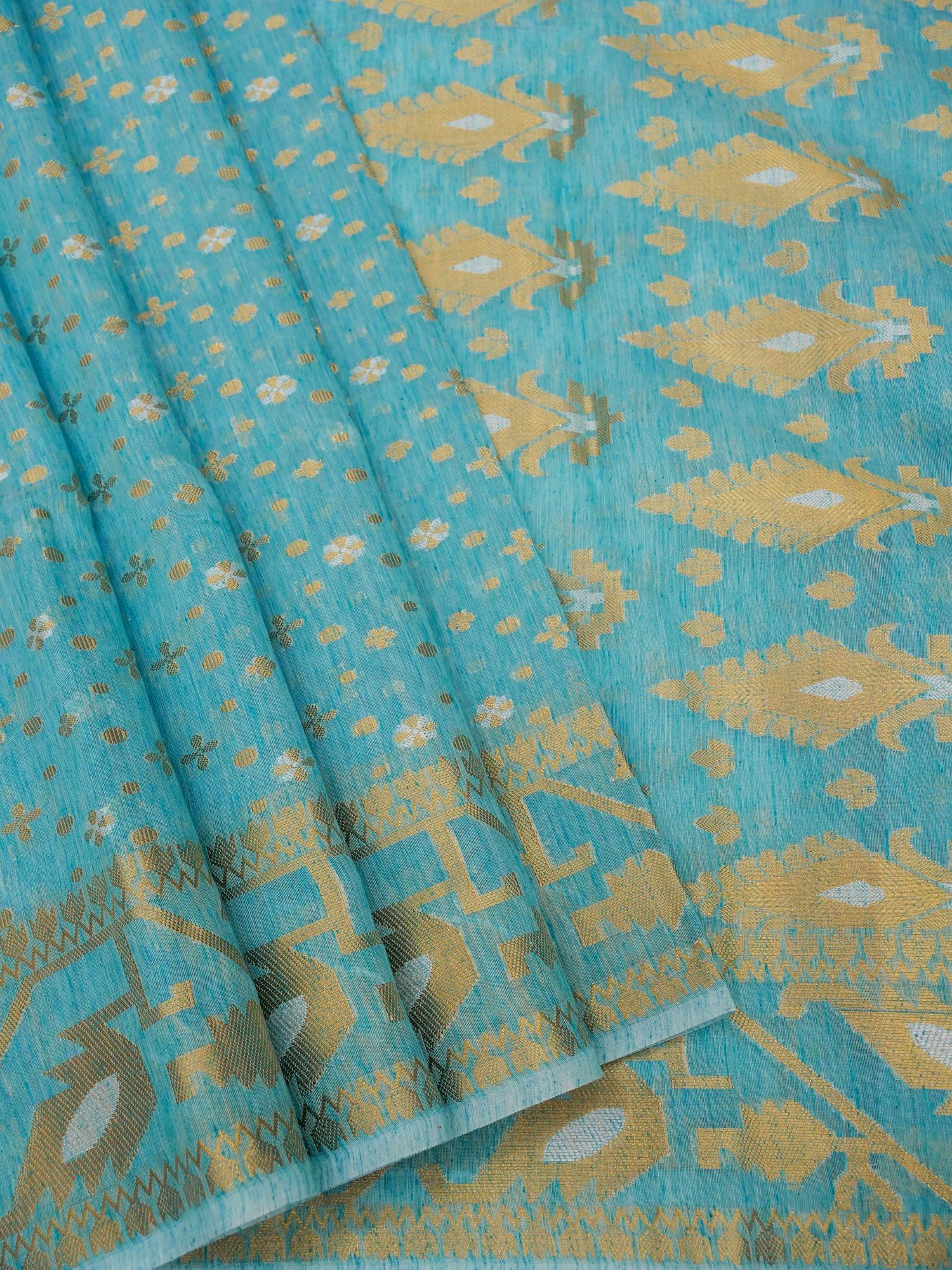This image features a vertically oriented textile tapestry composed of high-quality fabric in a beautiful light blue or turquoise color. The fabric boasts intricate golden patterns with a sheen that catches the light. The tapestry consists of two separate but similar fabrics layered over one another. 

The main fabric, occupying the majority of the image, is adorned with a diamond-shaped pattern. These diamonds feature textured ridges on the left side, smoothing out towards the right, and are filled with corn husk-shaped motifs and surrounded by small three-leaf shapes. The second fabric, draped over the main one on the left side, showcases a gold, almost flame-like pattern at the bottom edge, encircled by a zigzag row of tulip-like flowers. Additional elements include gold crosses, spots, and filigree patterns accentuating both fabrics.

Overall, the cloth appears heavy-duty and meticulously crafted with a mix of abstract and floral imagery, providing a rich, ornamental look.